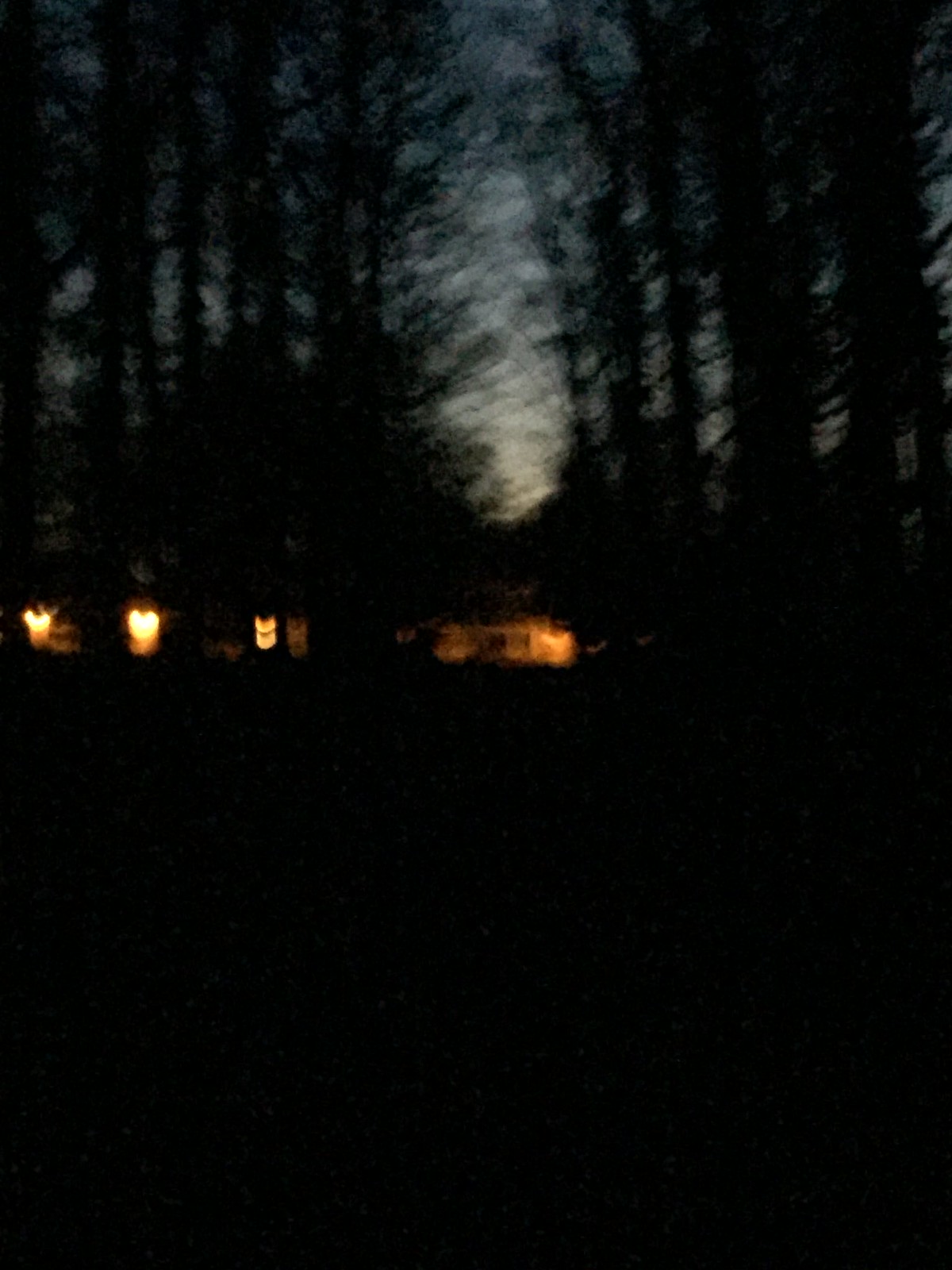In this very blurry and dark image, we observe a scene that appears to be set in a forested area. The top half of the image reveals a bluish-gray sky tinged with white, suggesting it could be either sunrise or sunset. This sky is partially obscured by the dark silhouettes of large trees surrounding the subject of the image. In the center, there is a distant, illuminated structure that most likely resembles a home. This structure emits a gold and orange glow, with a prominent rectangular light in the middle, indicating possible windows. Additional smaller, glowing spots can be seen to the left of the main light source, which adds to the impression of a house with multiple illuminated windows. The bottom half of the image plunges into absolute pitch blackness, reinforcing the sense of deep forest and solitude. The overall atmosphere conveyed is one of eerie tranquility, perhaps akin to encountering a lit cabin in the dense woods during the twilight hours.